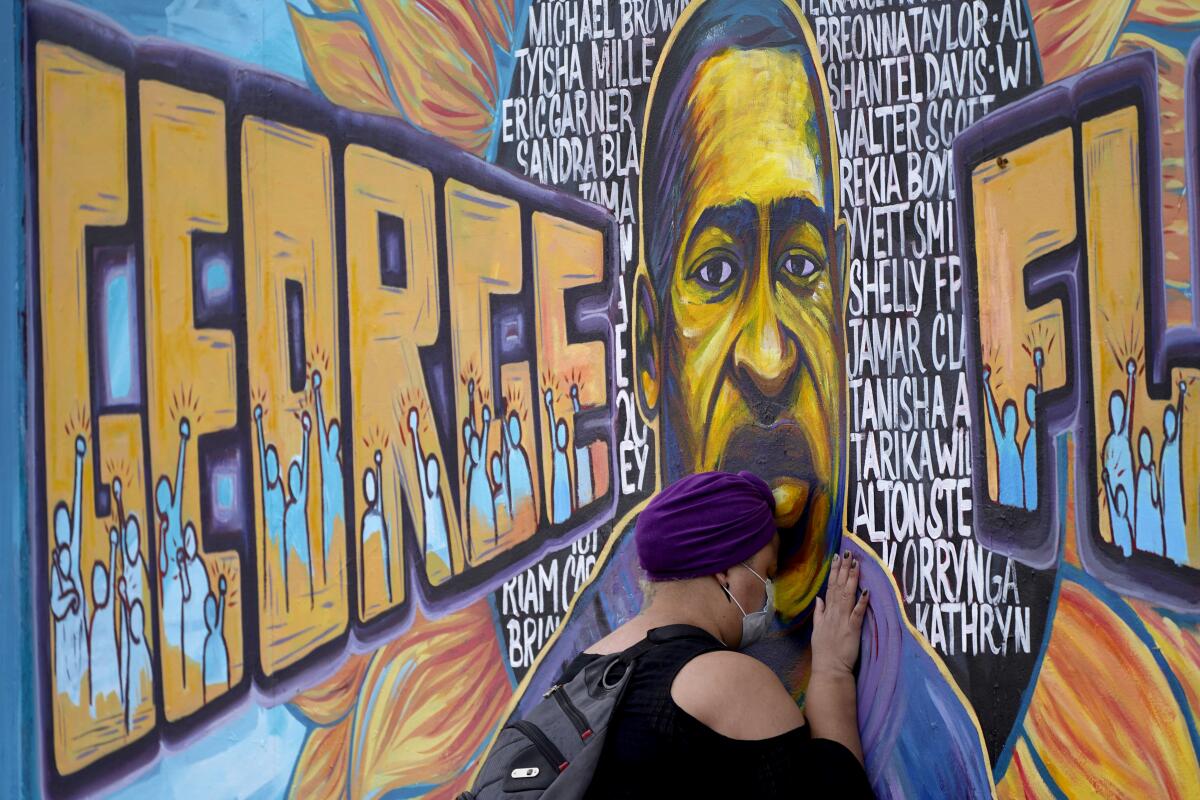The photograph depicts a vibrant mural honoring George Floyd, prominently featuring his portrait at the center. His face is surrounded by names of other victims of police violence, meticulously written in white letters that form a sunflower design. The mural’s colors are predominantly orange, blue, and black, with the name "George" in bold orange square font on the left side and the letters "F.L." on the right. George Floyd is illustrated wearing a purple hoodie, his image spanning the entirety of the wall or building. In front of the mural, a woman with a purple turban, a surgical mask, and a backpack is kneeling, her forehead pressed against the wall. This poignant scene likely reflects the period of the COVID-19 pandemic, encapsulating a moment of solemn reflection and tribute.